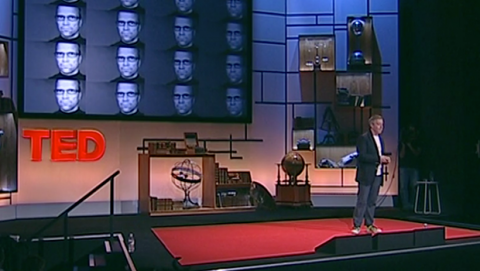The image captures a moment from a TED Talk taping. In the foreground, a man stands confidently on a red carpeted stage, gripping a microphone. He is dressed in a black business casual jacket over a white t-shirt, paired with gray slacks and white shoes. Directly behind him is an arrangement of various equipment, including speakers positioned at the edge of the stage, ensuring he can hear himself. 

Dominating the background is a massive screen showcasing a collage of the man's headshots, arranged in a grid of four rows and four columns, making a total of 16 images. Beneath the collage, the bold red letters "TED" stand out prominently. The stage setup also includes a set of shelves with a globe and possibly a sculpture, serving as part of the backdrop. To the man's right are stairs leading off the stage, and a stool situated off to the wings, adding to the set's casual yet professional atmosphere.